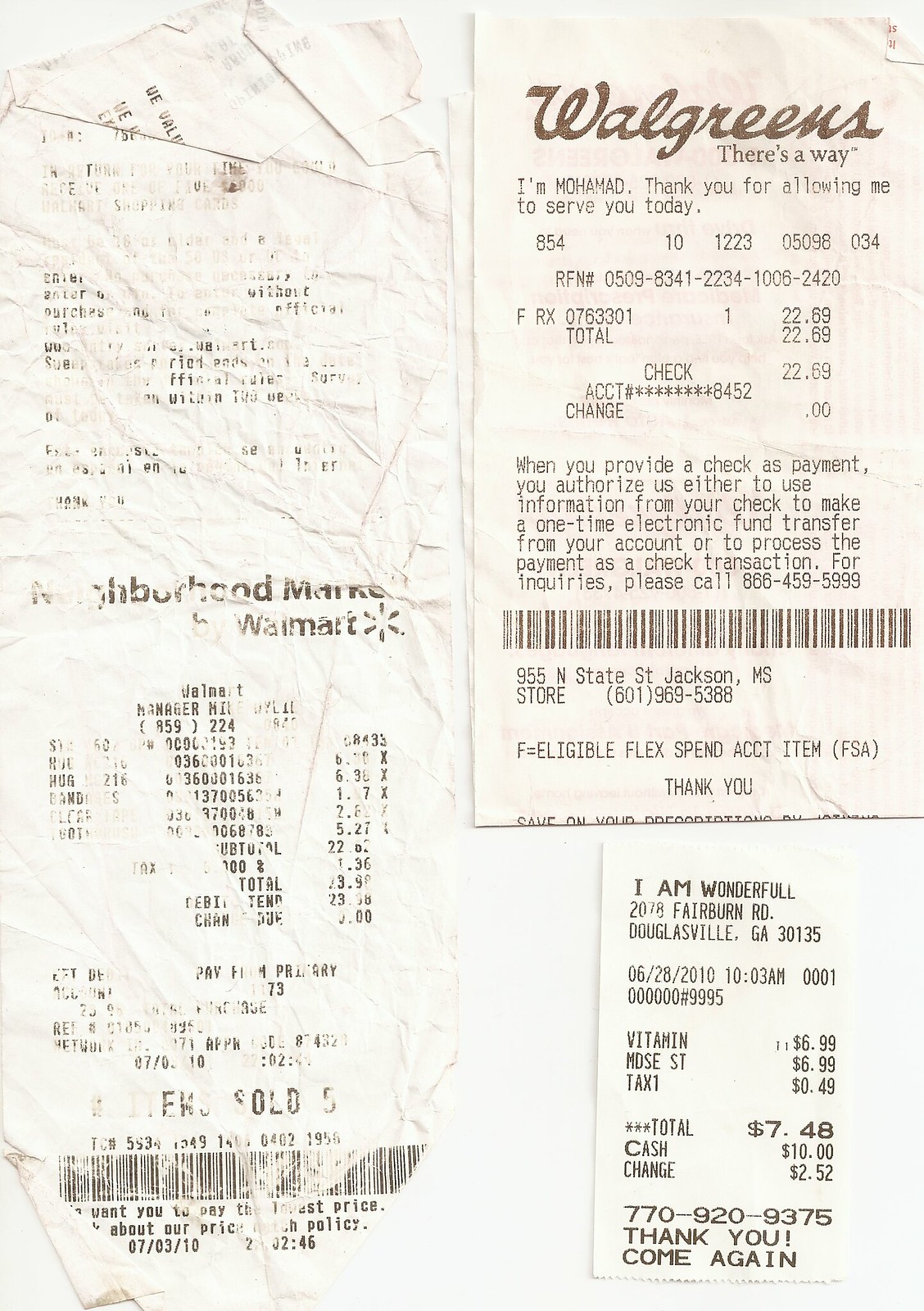This vertically-oriented color scan depicts three receipts arranged against a monochromatic backdrop. On the left, a lengthy Walmart receipt, heavily creased and worn, extends downward with most of the text faded and illegible. To the right of the Walmart receipt is a partially folded Walgreens receipt, visible at the top and right-hand corner. Despite minor creasing, the Walgreens logo and header are discernible. In the bottom right corner, a small, pristine receipt floats with the uplifting message, "I am wonderful." The image predominantly features shades of black, white, and grayscale, emphasizing the stark contrasts and details of the receipts’ wear and tear.